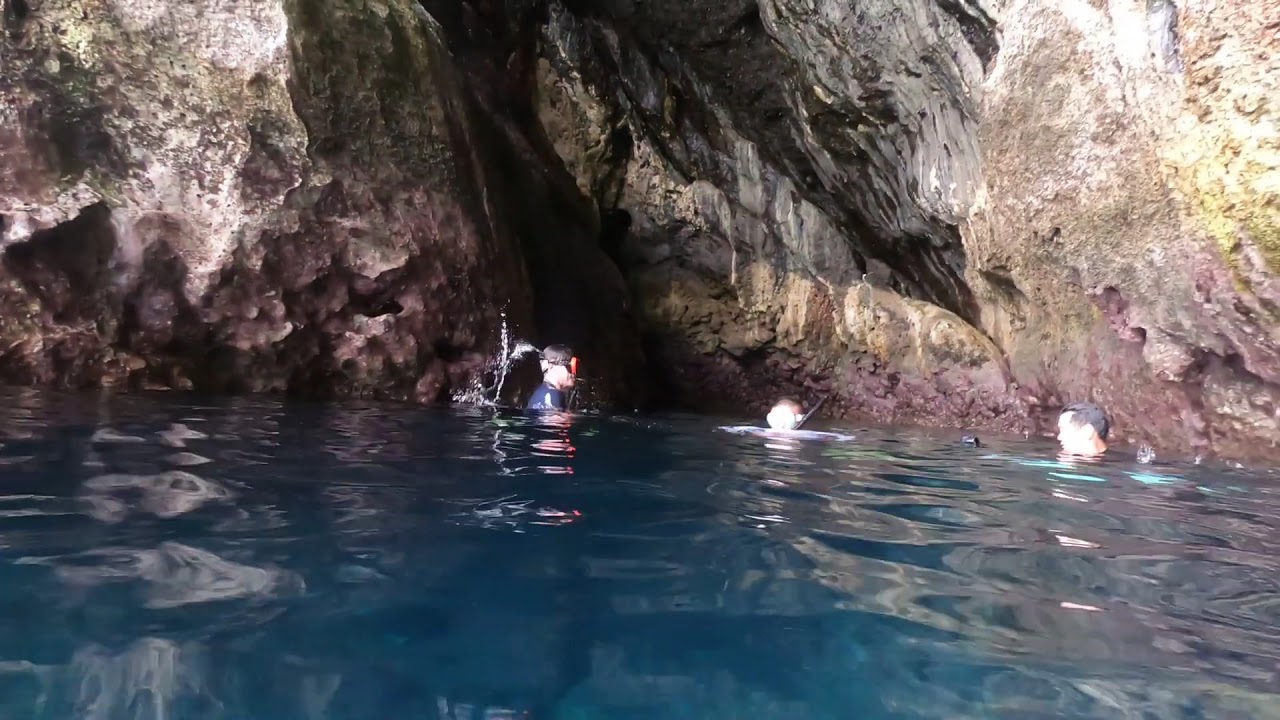In this captivating image, we see a serene outdoor setting featuring three people engaged in snorkeling within a calm, aquamarine body of water, surrounded by imposing, weather-worn rock walls. The scene is likely shot in the middle of the day inside a cavern or a mountain cove. The rough, natural rock formations, stained with shades of bleached white, darker browns, yellows, and greens, provide a striking backdrop. At the center of the image stands a trio consisting of two adult men and a child. The child, positioned in the middle, wears goggles and a snorkel, immersed in the water. The man on the left, slightly elevated, appears to be exhaling water through his snorkel, with orange goggles adorning his face. On the right, another man is seen with his snorkel removed, seemingly cleansing it in the tranquil water. This vivid composition captures a moment of exploration and interaction in a picturesque natural aquatic environment.